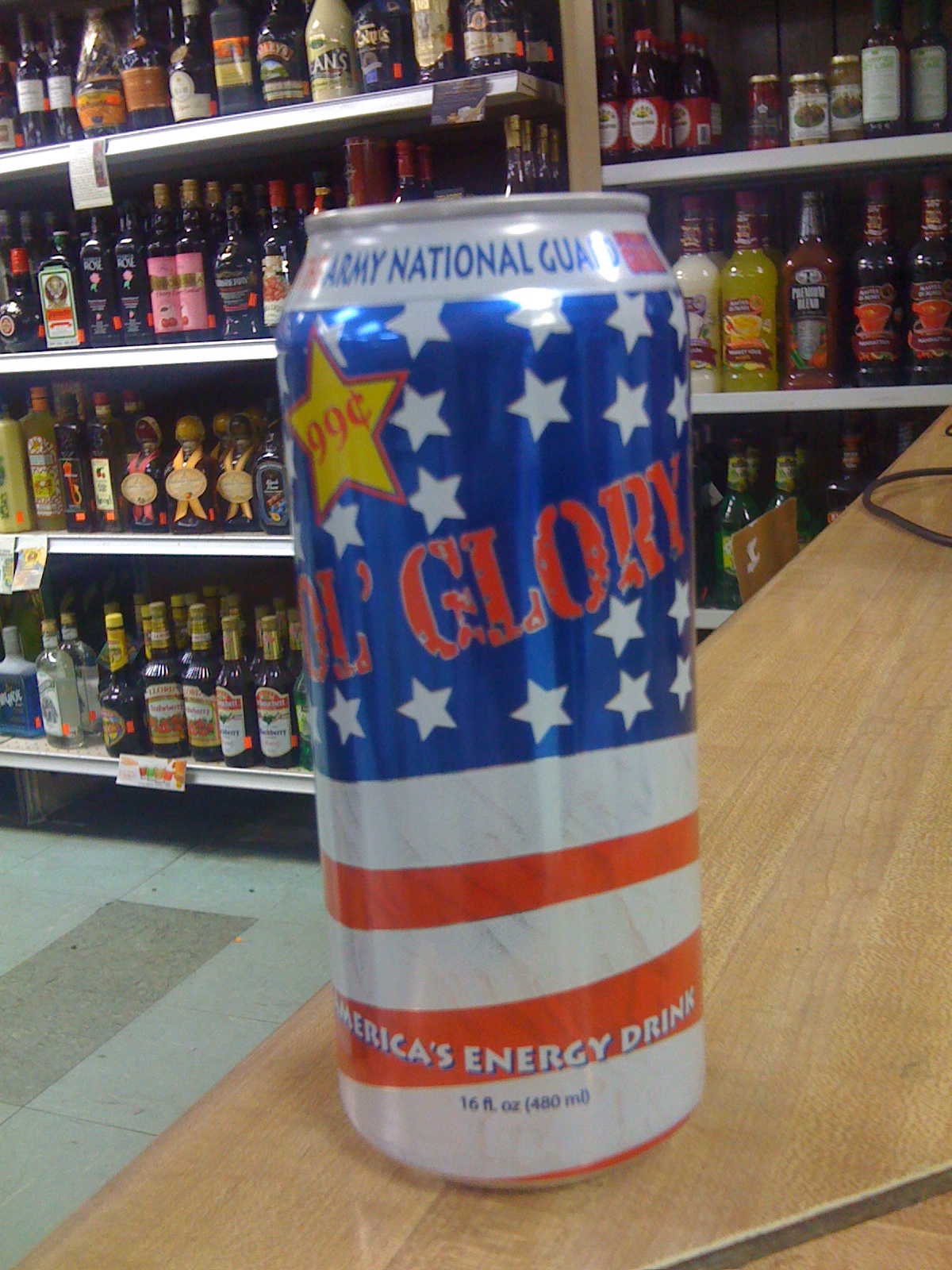The color photograph showcases a can of a drink prominently displayed on a long wooden countertop, positioned towards the right corner where a pin is also visible. The can, labeled "Old Glory," is designed with an American flag motif, featuring a blue background with white stars and red and white stripes. It prominently states "Army National Guard" at the top rim, declaring itself "America's Energy Drink." A golden star on the can indicates the price, 99 cents. The drink is 16 fluid ounces or 480 milliliters in volume. In the background, the scene is dominated by shelves stocked with various liquor bottles in assorted colors, indicating that the setting is a liquor store.